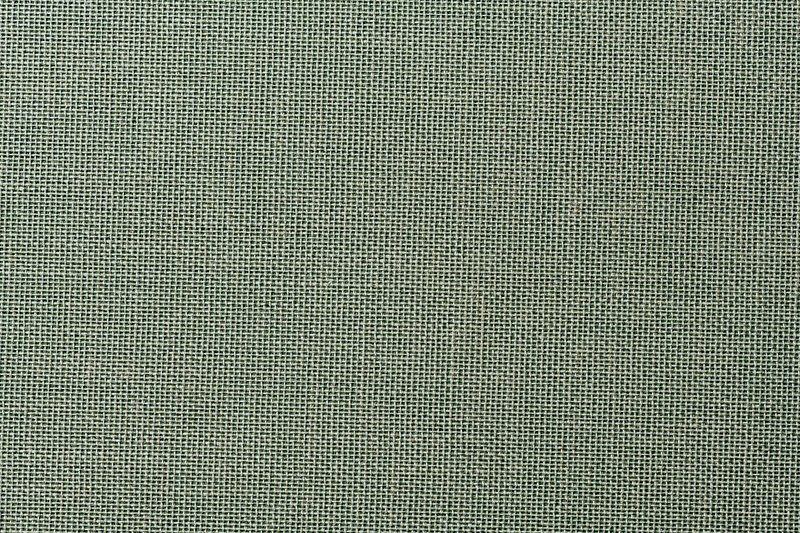This image is a highly detailed, up-close photograph of a piece of burlap or similar woven fabric material. Displayed in a square format, the image captures the intricate textures created by the intersecting threads, forming tiny, textured boxes. The fabric is laid out flat, unwrinkled, and appears to have been ironed or steamed, ensuring a smooth presentation. The color of the material is a blend of light tan, green, and gray, with subtle shadings of white interspersed. The fabric occupies the entire frame, approximately 4 inches by 5 inches, with no additional elements, text, or context provided to indicate its purpose or future use. The setting remains plain and unembellished, focusing solely on the detailed texture and weave of the fabric itself.